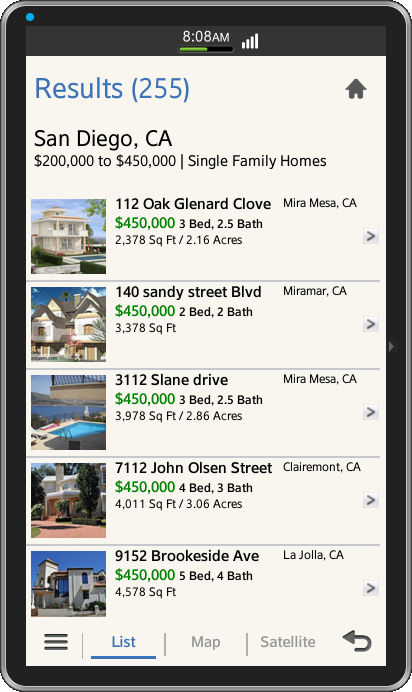The image displays a digital device, possibly a tablet or smartphone, open to a real estate search results page. At the top of the screen, the search has yielded 255 results, indicated in brackets, with the search criteria being "SanDiego.ca" and a price range spanning from $200,000 to $450,000 for single-family homes. On the visible portion of the screen, five property listings are displayed:

1. **112 Oak Glenard Clove, Miro Mesa, CA**
   - Price: $453,000
   - Bedrooms: 3
   - Bathrooms: 2.5
   - Additional details available at the bottom of the listing.

2. **140 Sandy Streak Blvd, San Diego, CA**
   - Price: $450,000
   - Bedrooms: 2
   - Bathrooms: 2

3. **3112 Slane Drive, San Diego, CA**
   - Price: $450,000
   - Bedrooms: 3
   - Bathrooms: 2.5

4. **7112 John Olsen Street, San Diego, CA**
   - Price: $450,000
   - Bedrooms: 4
   - Bathrooms: 3

5. **1952 Brookside Avenue, San Diego, CA**
   - Price: $455,000
   - Bedrooms: 5
   - Bathrooms: 4